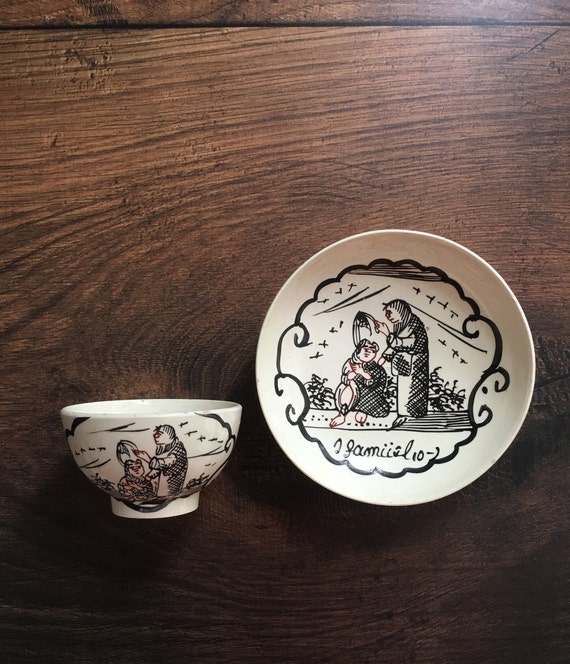This photograph showcases a white teacup and saucer set, placed on a wooden table. Both the teacup and saucer feature matching black ink illustrations and designs. The overhead view reveals that the drawings depict an intimate scene: a taller woman stands as she helps a shorter woman, possibly indicating a familial relationship, such as a grandmother assisting a sister or relative. The taller woman holds a pair of scissors to the tips of the shorter woman's extraordinarily long hair, suggesting she is about to cut it. Surrounding them, the saucer features an ornate circle around its edge, while the bottom part of the saucer includes text that reads "familio," hinting at the theme of family. Additionally, the background of the illustrations includes elements like trees and the sky, adding to the depth of the design. The teacup mirrors this same detailed scene on its side, further emphasizing the close connection between the two pieces in this set.